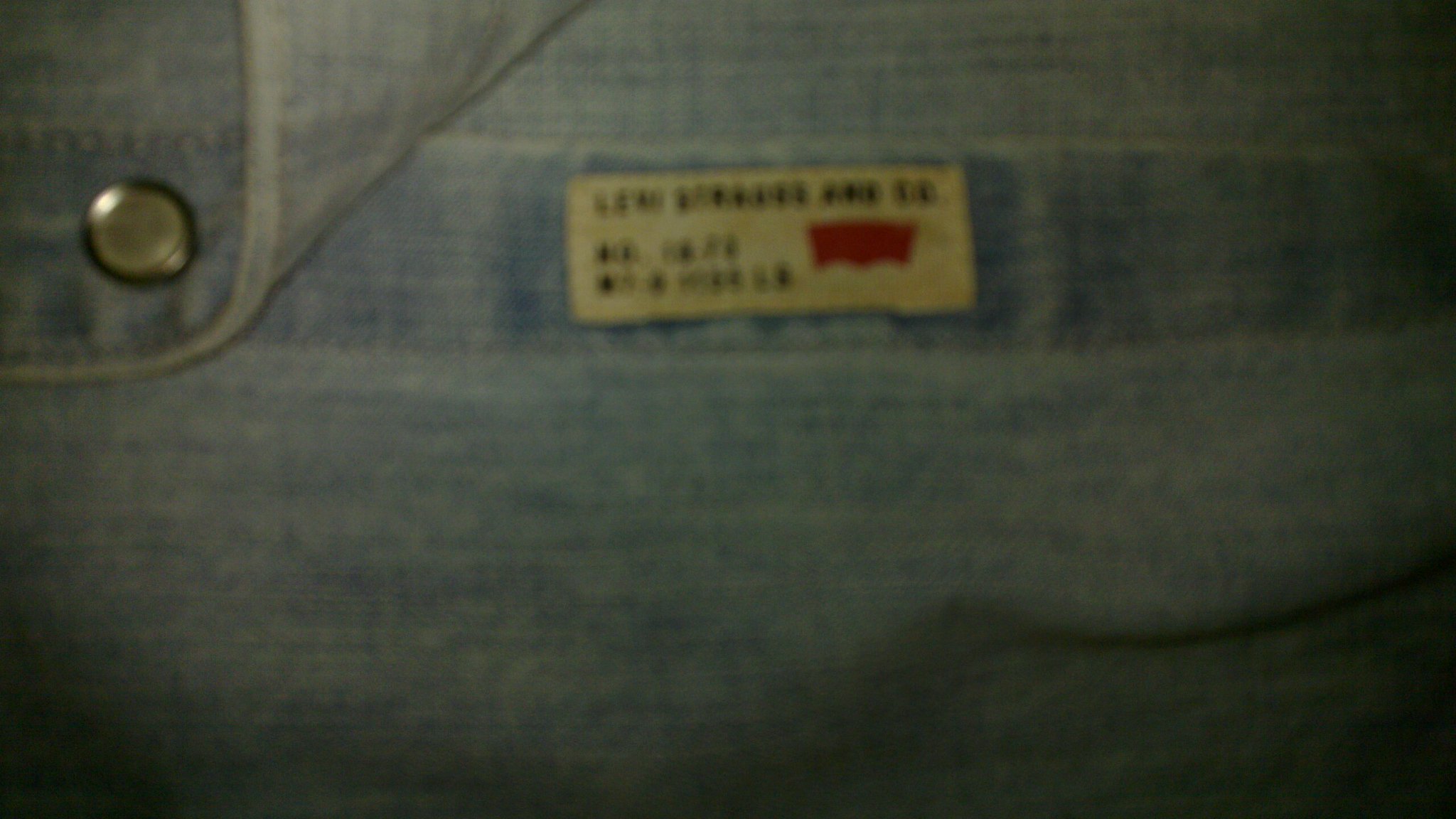The image is a close-up view of a blue denim fabric, likely from a piece of clothing such as jeans or a shirt. The fabric appears faded and features a partially folded flap at the top left corner, secured by a small silver button. Above this button, stitching is visible. Below the flap, there is a horizontally rectangular white tag with indistinct black text and a red symbol that resembles a Levi's logo. The fabric exhibits striations running horizontally across it, and a crease can be seen at the bottom left. The image is somewhat blurry and poorly lit, casting a yellowish hue over the scene, with the bottom and right sides being particularly dark.